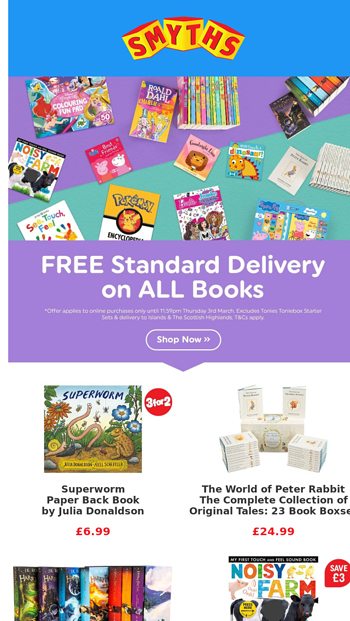The image is a screenshot of an online bookseller's webpage. The top section features a light blue stripe running from the upper left to the upper right, with a central logo that reads "SMYTHS." Below this, there is a vibrant display of children's books set against a purple and green background, showcasing titles such as "Roald Dahl," "Noisy Farm," "Pokemon," and "Coloring Fun Pad."

Underneath this main banner, a purple stripe includes text stating "Free standard delivery on all books," with an unreadable font next to it and a clear, clickable button labeled "Shop Now" followed by two forward arrows.

The next section of the webpage has a white background and is organized into two columns. Each column displays two items. The top-left item in this section is "Superworm" by Julia Donaldson, a paperback book priced at £6.99 with a red tag indicating a "3 for 2" offer. To the right of it, there's "The World of Peter Rabbit: The Complete Collection of Original Tales" – a 23-book set priced at £24.99. Each listing includes images of the respective books.